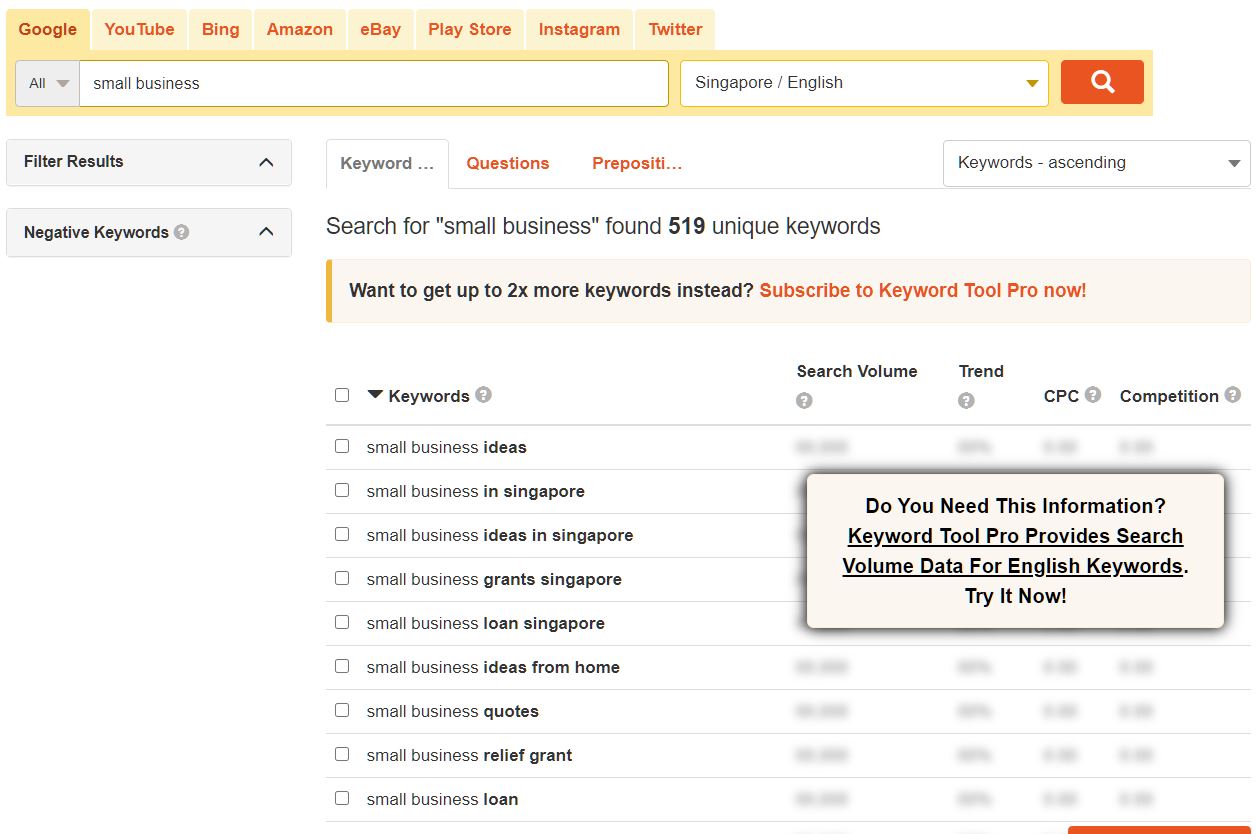The image depicts a busy webpage with multiple tabs open at the top, with "Google" as the active tab. Additional visible tabs include YouTube, Bing, Amazon, eBay, Play Store, Instagram, and Twitter. In the Google search field, the text "small businesses" is entered, and the interface displays "Singapore / English" next to the search bar. The search button is noticeable with its orange color and a white magnifying glass icon.

The search results interface offers options to filter results and navigate keywords using an upward caret symbol. The main exploration area includes "Keywords," "Questions," and "Prepositions," with the "Keywords" section currently selected and displayed in gray, while the other sections are highlighted in orange. The search phrase "small businesses" returned 519 keyword results.

A promotional message beneath the keyword count entices the user to subscribe to "Keyword Tool Pro" for access to up to two times more keywords, with "Subscribe" prominently displayed in orange. The list of keywords shown includes terms like "small business ideas," "small business in Singapore," "small business grant Singapore," "small business loan Singapore," "small business ideas from home," "small business quotes," "small business relief grant," and "small business loan."

Additional details like search volume trends, CPC (Cost Per Click), and competition levels are present but grayed out, accompanied by a message highlighting the advantages of the "Keywords Tool Pro" service. This message invites the user to try the tool for comprehensive search volume data for English words.